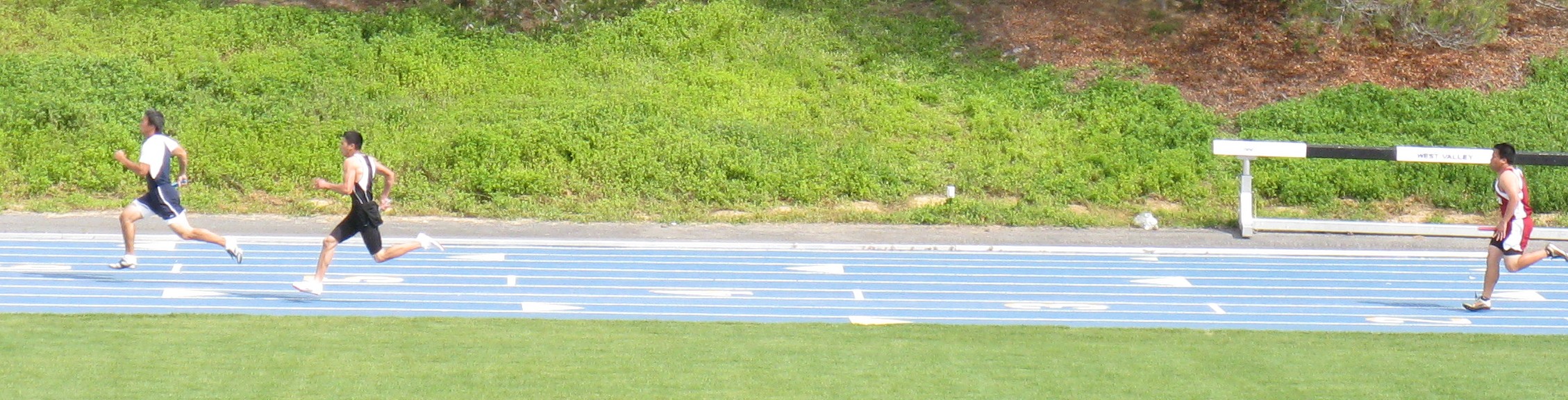In this detailed horizontal photograph, approximately an inch and a half high by seven inches wide, three men are captured running on a light blue track marked with white lines. The runner on the right wears red and white shorts and a matching sleeveless top, while his white sneakers contrast with the blue of the track. To the left, another man sports black shorts and a likely black and white top, flanked by a third runner in blue shorts with white detailing and a coordinating blue and white top. The image composition features green grass stretching across the foreground, while the track runs horizontally, bordered by a slightly elevated area of green shrubs and various vegetation on the other side. A noticeable detail is a black and white striped barrier set against the track’s side and a hurdle positioned on the upper right, not in use but adjacent to the lone runner on the right. The scenery behind the track ascends on an incline, showing patches of brown dirt among the greenery.